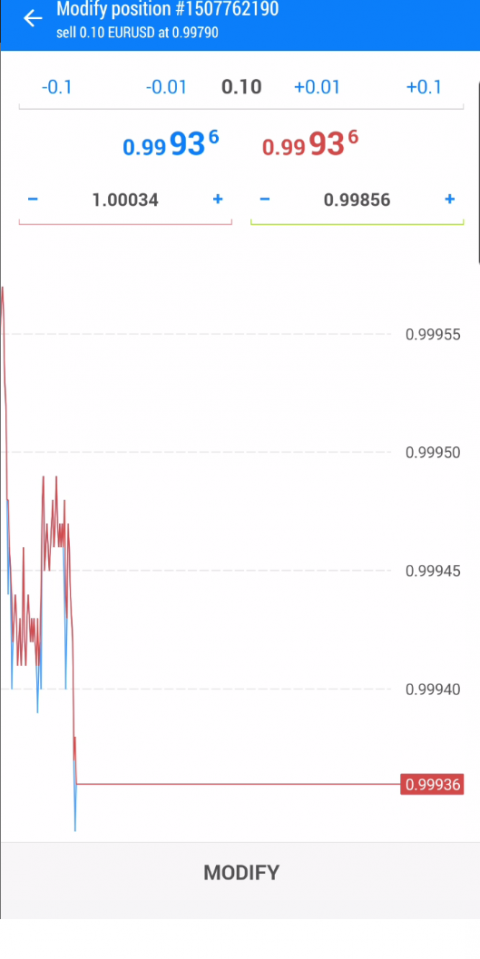The image features a detailed, data-rich graphical analysis set against a clean, white background. At the top, there is a prominent blue box containing an arrow pointing left with the text: "Modify Position Number 1507762190, Cell 0.10, Eloroust at 0.99790." 

In the center of the image, a series of numerical values are displayed in various colors, showcasing both positive and negative increments. Specifically:

- Negative values such as -0.1 in blue and -0.01 in blue.
- Neutral value 0.10 in black.
- Positive values such as +0.01 in blue and +0.1 in black.

A distinctive line is present in the middle, associating multiple numerical data points:
- 0.99 with a superscript "6" to the right,
- 93 as another notation.

Towards the right, in red, repeated values include:
- 0.99 with a superscript "6",
- 93.

Further along, a sequence of intricately detailed decimals is displayed, capturing very fine variations:
- 1.00034 in blue with a blue minus and blue plus nearby,
- 0.99856 in blue with a blue plus,
- A black dividing line on the outer edge with these values outlined in black,
- Other lines following detailed decimals such as 0.99955, 0.99950, 0.99945, and 0.99940.

On the left side, a set of red and blue lines ascend and descend, intersecting with the detailed measurement lines, indicating dynamic change. At one point, the values peak just above 0.99955 before descending.

At the bottom, there is a concluding red line coupled with a red box containing the value 0.99936, alongside a smaller blue box labeled "Modify." This juxtaposition of colors and values within the structured graphical elements gives a comprehensive, albeit complex, visualization of the dataset in question.